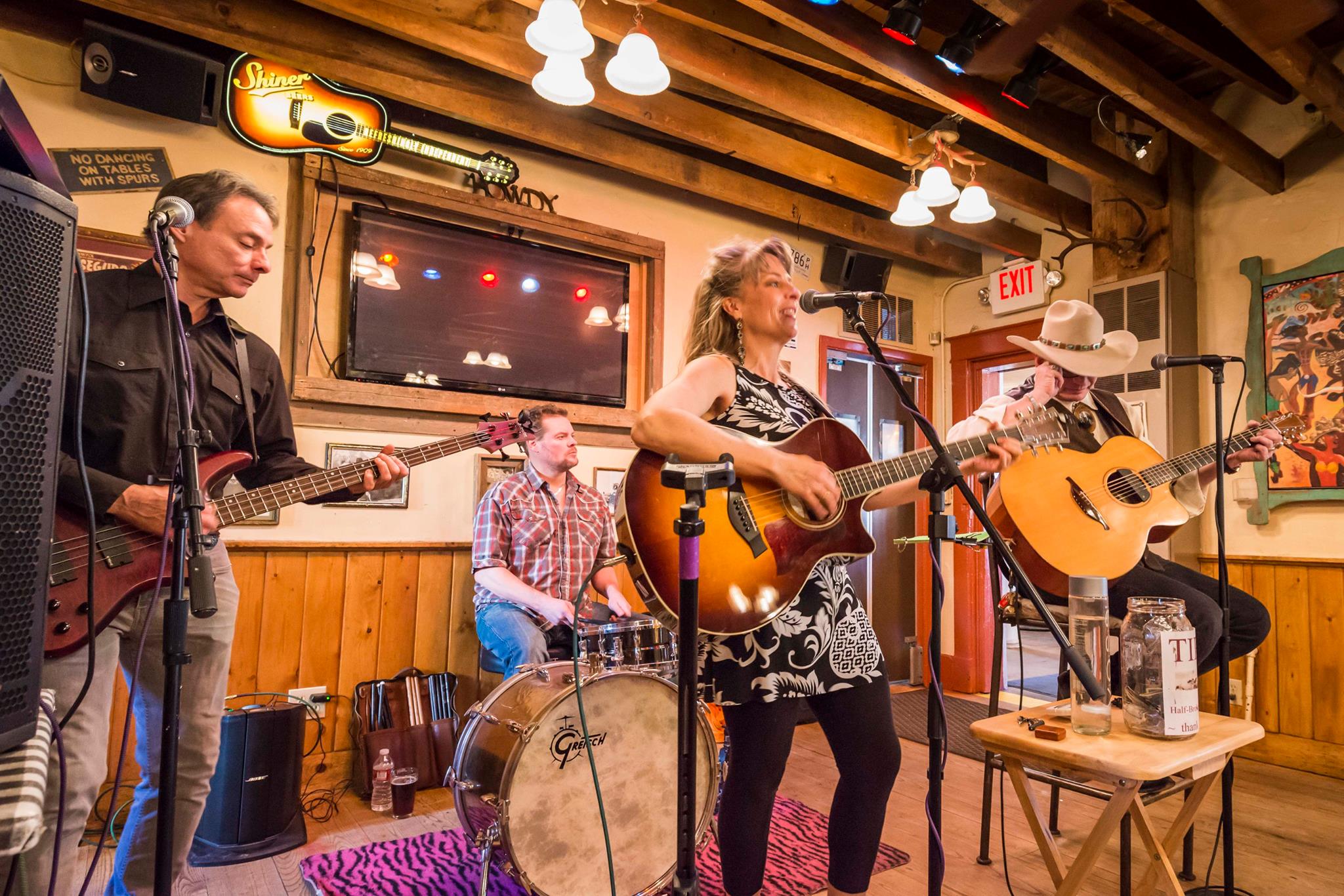This vibrant photograph captures a live performance at a rustic bar, characterized by its wooden panels and beams. Central to the image is a woman with grayish, dirty blond hair styled in a half ponytail. She is energetically strumming an acoustic guitar and singing into a microphone. She is dressed in a black and white floral tank dress paired with black stockings and stands on a distinctive pink and black zebra-style rug.

To her right, a man in a white shirt, black pants, and a brown vest sits on a stool, also playing an acoustic guitar. He completes his look with a cowboy hat and looks down at his instrument, a microphone poised in front of him.

The drummer is positioned behind and to the left of the woman, clad in a short-sleeve plaid shirt and blue jeans, his short brown hair visible as he plays the drums. To the far left, another male performer stands with a burgundy bass guitar. He sports a black button-down collared shirt and gray denim jeans, focused on the music with a microphone stand before him.

The cozy bar setting includes wooden panels on the walls and wooden beams on the ceiling, accented by hanging speakers and lights. A flat-screen TV is mounted on the wall behind the band, switched off, with a guitar hanging above it and a sign that reads "Shiner." A small wooden table between the central figures holds a clear jar for tips, adding to the intimate, folksy atmosphere of the scene.